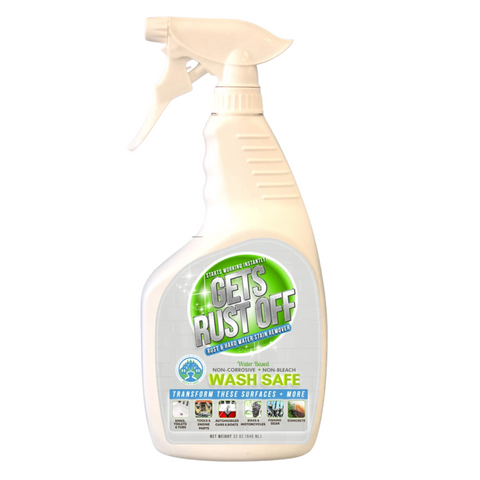This is a detailed photograph of a beige cleaning spray bottle set against a white background. The bottle, viewed from the side, has a spray nozzle at the top which points to the left, featuring a handle that releases the cleaning liquid when pressed. The bottle's label has a light blue background with text that reads “Gets Rust Off” in a gray, silver-highlighted font. Below this, the label states “Wash Safe” and “Transforms These Surfaces,” accompanied by small pictures depicting various surfaces that the product can clean. The label also emphasizes the product’s non-corrosive and non-bleach properties. The design prominently features a green circular outline with lighter, almost white shading towards the center, adorned with white star circles at the bottom left.